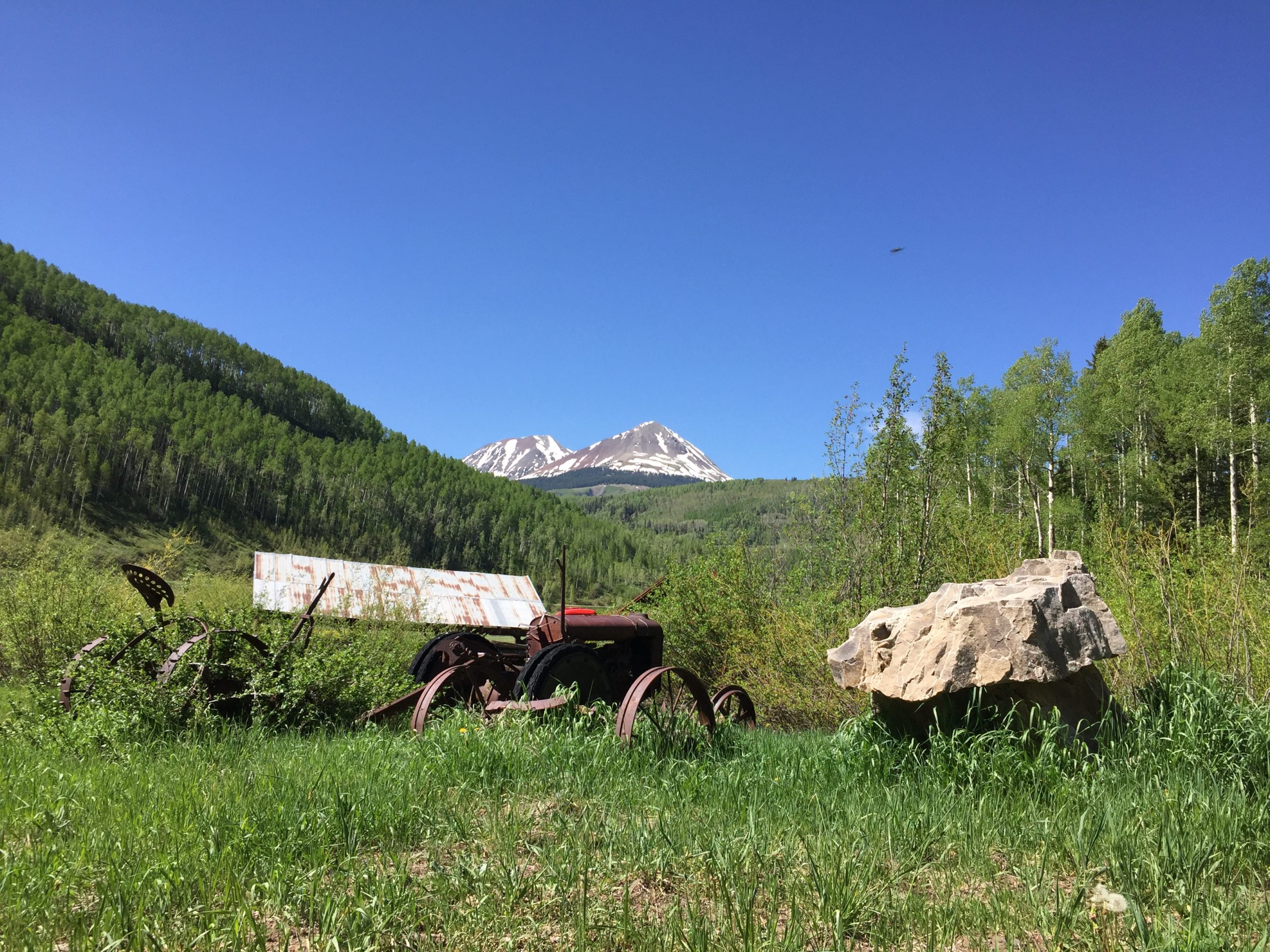This professionally taken outdoor photo captures an abandoned and rusted tractor, suggesting it hasn't been used in a long time, sitting in a green grassy valley with patches of brown soil and some overgrown weeds. The tractor, which might be as old as a lawnmower, features metal rims instead of rubber tires. To the right of the tractor, there's a large, jagged tan-colored boulder. In the background, rolling hills covered in dense trees lead up to distant snow-capped mountain peaks under a rich blue, cloudless sky. This picture is devoid of people, animals, movement, or any text, focusing purely on the serene yet static rural landscape.